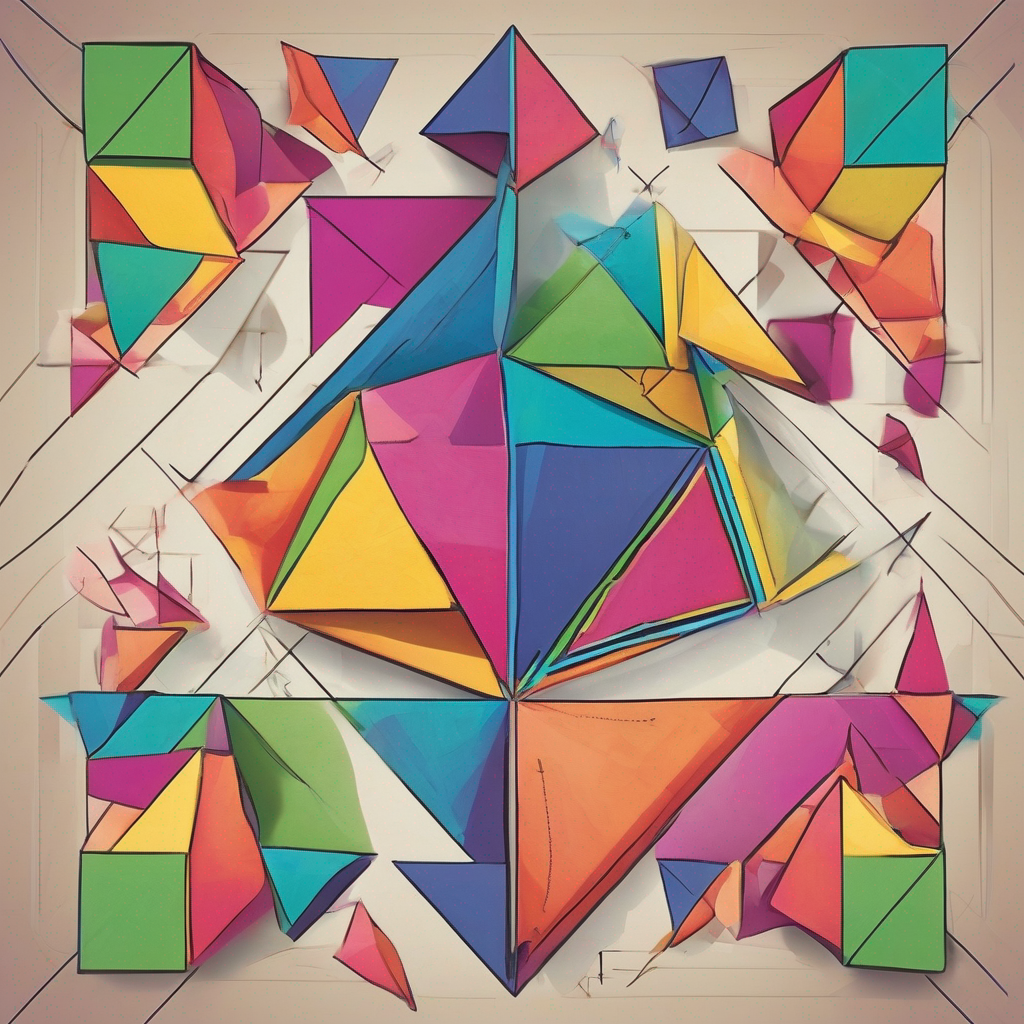This image showcases a dynamic and intricate painting rendered in a geometric style. The focal point is a diamond shape that appears to have exploded into a myriad of pieces, creating a sense of chaotic splendor. These fragmented pieces exhibit a vibrant array of colors including orange, fuchsia, indigo, violet, turquoise, teal, green, yellow, gold, pink, and various shades of rose, all delineated by stark black lines. The explosion of colors is contained within a seemingly box-like space, suggested by precise geometric lines that impart a sense of dimension and structure at each corner. The surrounding space or "room" is painted in a contrasting brown hue, which further accentuates the vivid color burst at its center. The interplay of colors and shapes creates a visually stimulating and intriguing composition that captures the viewer's attention.